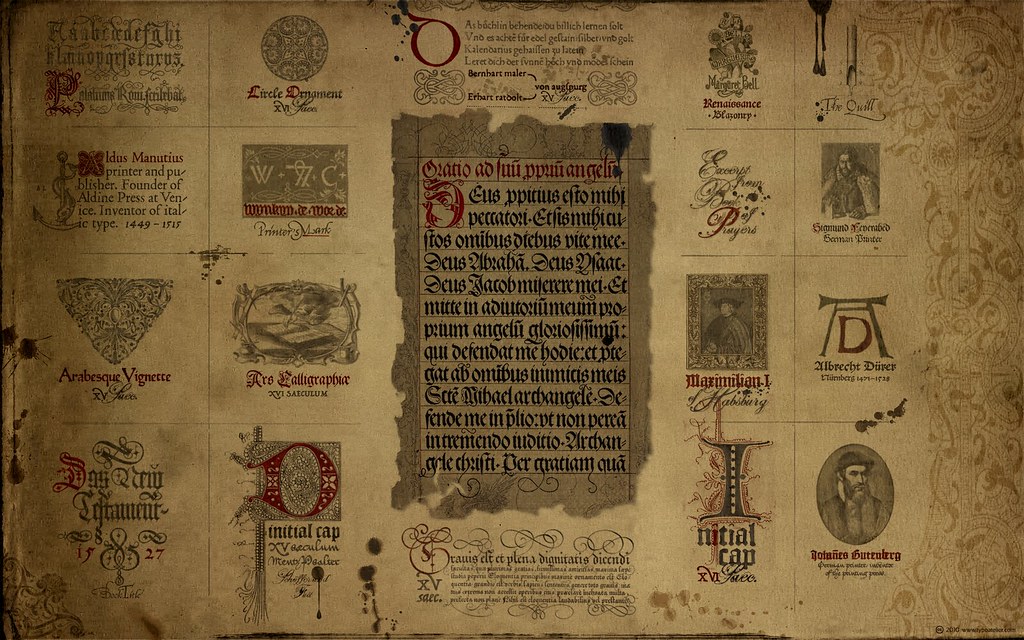The image depicts an old, light brown piece of parchment adorned with an array of intricate details. In the center, there is striking, stylish text written in black and red colors, resembling an old-world script in a foreign language. Surrounding this central text are numerous illustrations, including portraits of people, and geometric designs such as circles and triangles, all rendered in gray. The text accompanying these drawings is also in black and red, meticulously scattered across the parchment.

Notably, the page is sectioned off into distinct areas by lines, each containing a mix of text and illustrations, some resembling old-time crests or names, arranged in rows. On the right-hand side, there is a beautifully curved border design, adding to the antique appearance of the paper. The parchment also features black splotches and stains, heightening its old and historic look. Despite the language barrier, it's evident the document is designed to convey a sense of aged authenticity and elaborate documentation.